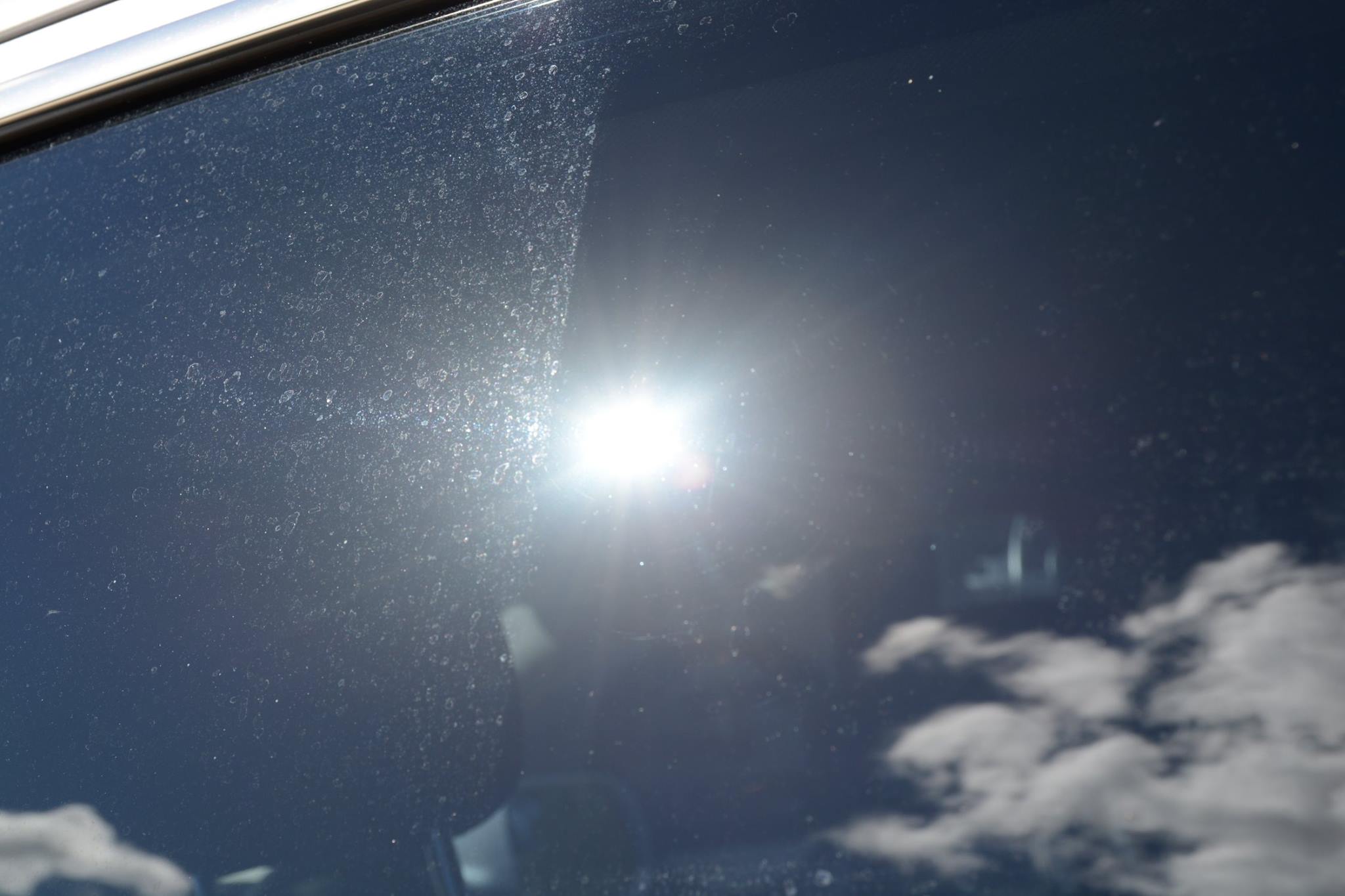This rectangular photograph captures a striking reflection in what appears to be the window of a car, with the frame of the car possibly visible in the top left corner. Dominating the center of the image, a brilliant sun shines intensely, creating an explosion of light that is captured on the glass surface. Surrounding the sun are fluffy white clouds, contrasting against what seems to be a dark blue sky in the reflection. The left side of the window bears noticeable dirt and dust spots, resembling beads of water that have dried, forming a clear distinction from the cleaner right side. This segmented appearance suggests it might be a partially cleaned window, as if someone was in the process of cleaning and paused, leaving one half significantly clearer than the other. The reflection of the sky and elements on the cleaner right side of the window is much more vivid and unobstructed, while the left side remains murky and spotted.